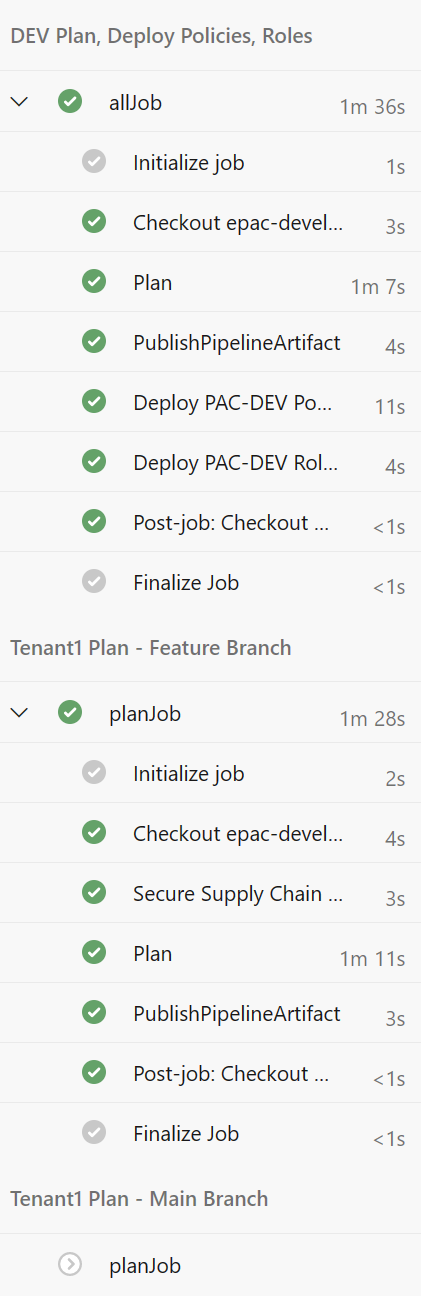This screenshot from a cell phone displays a detailed interface of a software application, specifically focusing on task and policy deployment management. The header of the screen reads "DED Plan" with sub-headings "Deploy Policies and Roles." Below these headings, the screen shows the comprehensive "All Jobs Menu," which provides a list of various tasks available within the application. These tasks include:

1. Initialize Job
2. Checkout
3. EPAC Develop Plan
4. Publish Pipeline Artifact
5. Deploy PACDEV co
6. Deploy PACDEV Role
7. Post Job Checkout
8. Finalize Job
9. Tenant Plan Feature
10. Branch Plan Job
11. Initiate Job
12. Checkout EPAC Develop 
13. Secure Supply Chain Plan
14. Publish Pipeline Artifacts
15. Post Job Checkout
16. Finalize Job
17. Tenant Plan Main Branch
18. Plan Job

Each task is designed to manage specific parts of the deployment and development process effectively. The interface aims to streamline the workflow of progressing from planning to deployment, showcasing how each phase is segmented into distinct, manageable units.